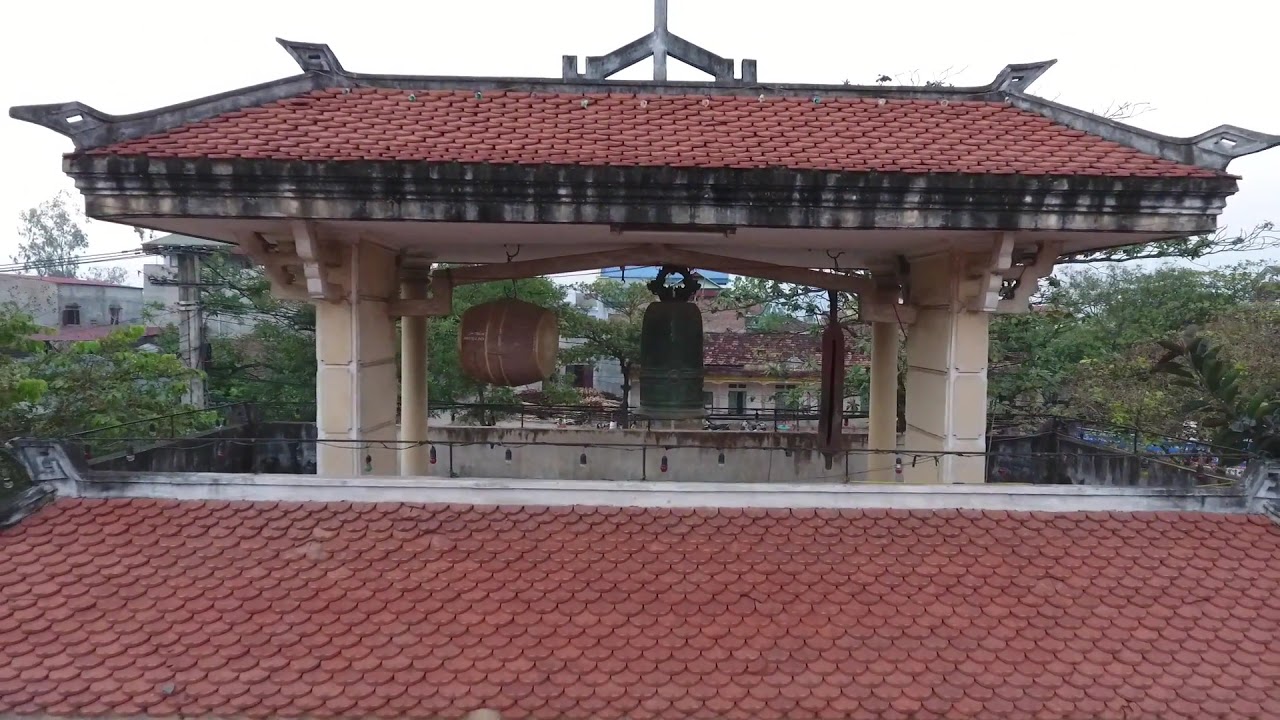The image captures the roof of an Asian-style building or temple, possibly situated in a town square or similar environment, given the architectural hints. At the center of the image, there is a bronze or light green copper bell hanging from a wooden beam. To the left of the bell, there is a barrel-shaped drum. This bell and drum setup is supported by two cement pillars. The roof itself features terracotta rounded tiles, and just below, another angled roof with similar terracotta tiles runs along the bottom of the image.

Surrounding and overhanging the roof are numerous green plants and tree branches, creating a sense of lush foliage enveloping the structure. In the distance, beyond the foliage, some run-down grey and terracotta buildings are visible. These buildings, alongside some electrical lines, complete the distant background. The sky above is clear, adding to the serene atmosphere of the scene. The elevated vantage point of the photograph suggests it was taken from a high position, perhaps another building nearby.